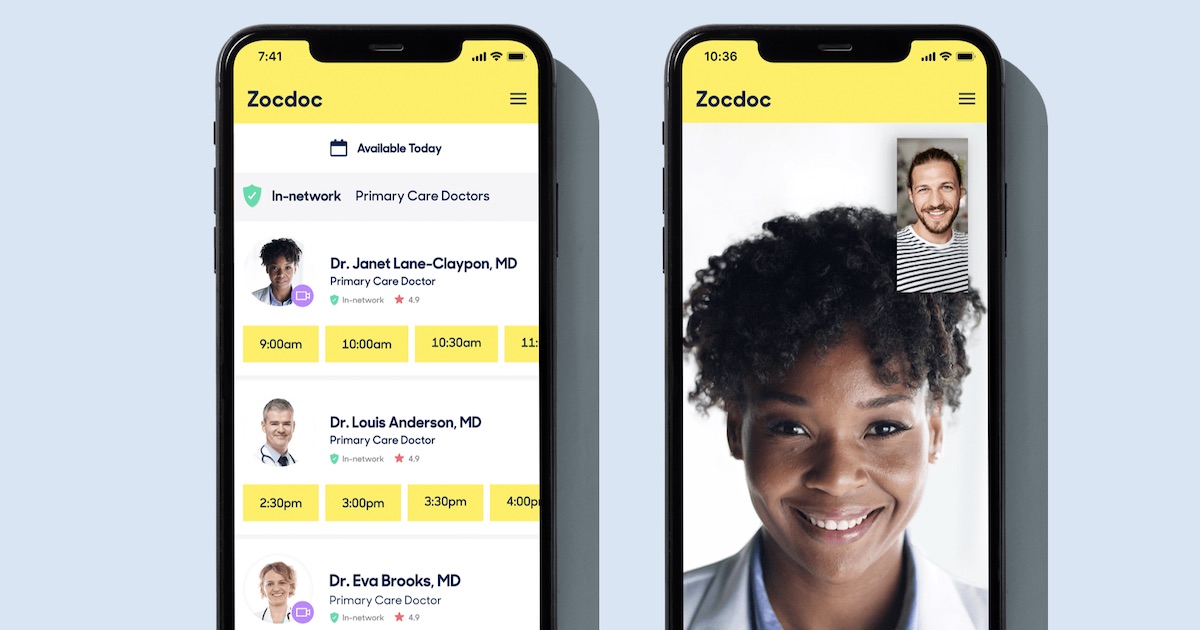The image showcases a website featuring two mobile phone screens displaying the ZogTalk app. On the left screen, the ZogTalk interface is visible, demonstrating how the app lists primary care doctors. The title "ZogTalk" is prominently displayed at the top. Directly below, the text "Primary Care Doctors" is shown, indicating the network of available healthcare professionals. The interface displays three doctors: a Black woman, a white man, and a white woman, each accompanied by their available consultation times, which vary from night to afternoon and evening. Next to each doctor's photograph, their names and the title "Primary Care Doctor" are clearly indicated.

The right screen appears to depict a mock-up of a phone consultation within the ZogTalk app. It features a large image of the doctor's face and a smaller image of the patient on the right side, simulating the interaction during a virtual visit. This detailed visualization effectively demonstrates the functionalities and user interface of the ZogTalk mobile application.